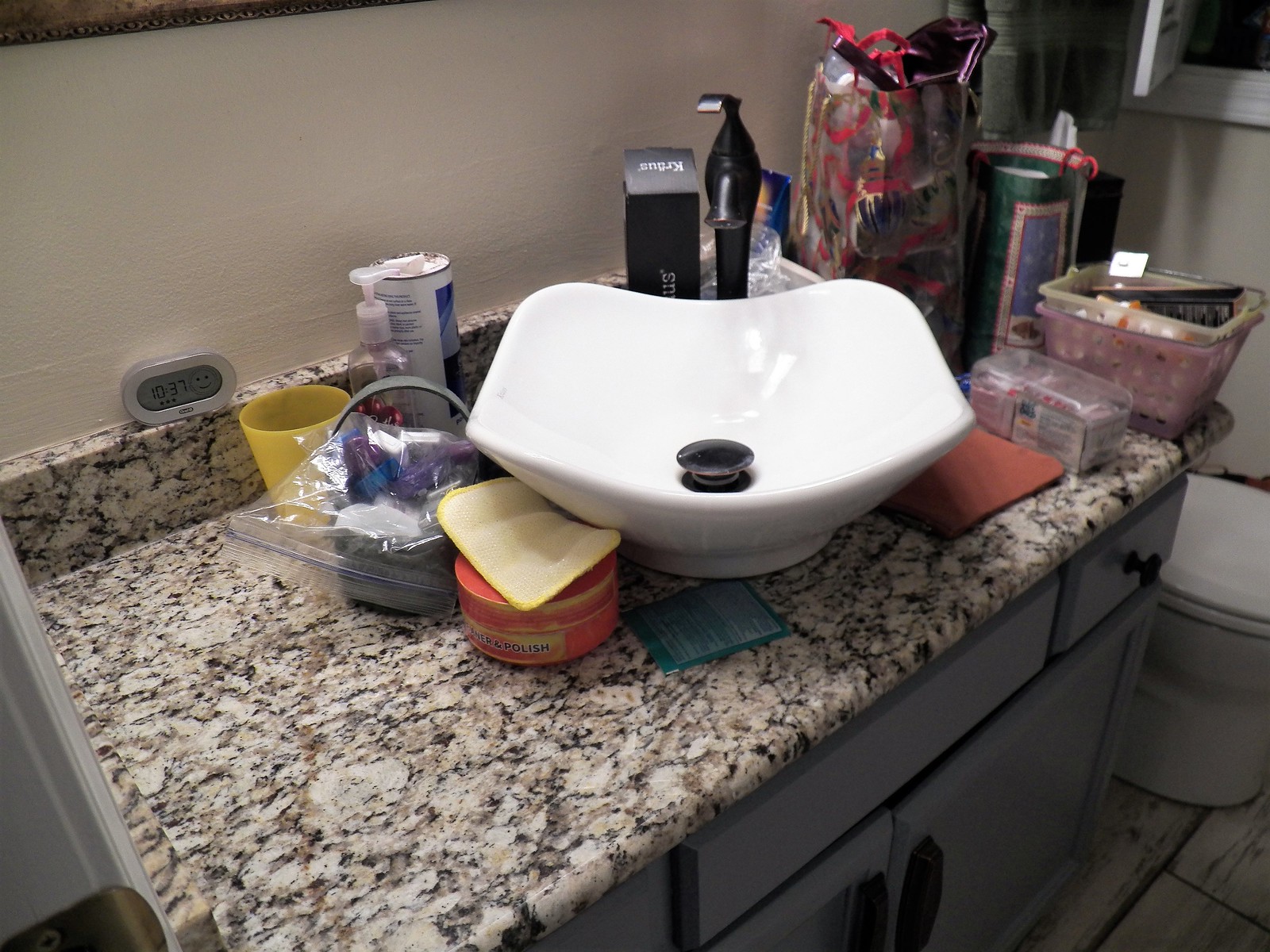In this traditional photograph, a cluttered bathroom is captured in detail. At the center of the image, a white sink is mounted on a speckled stone counter. Flanking the sink on both sides are numerous bathroom products, haphazardly stacked and scattered, creating a disordered appearance. To the right of the counter sits a white toilet. The small, indecipherable text on some of the bathroom products suggests labels and instructions, yet it remains unreadable due to its size. The entire scene exudes a sense of everyday chaos, reflecting the untouched state of a well-used bathroom.